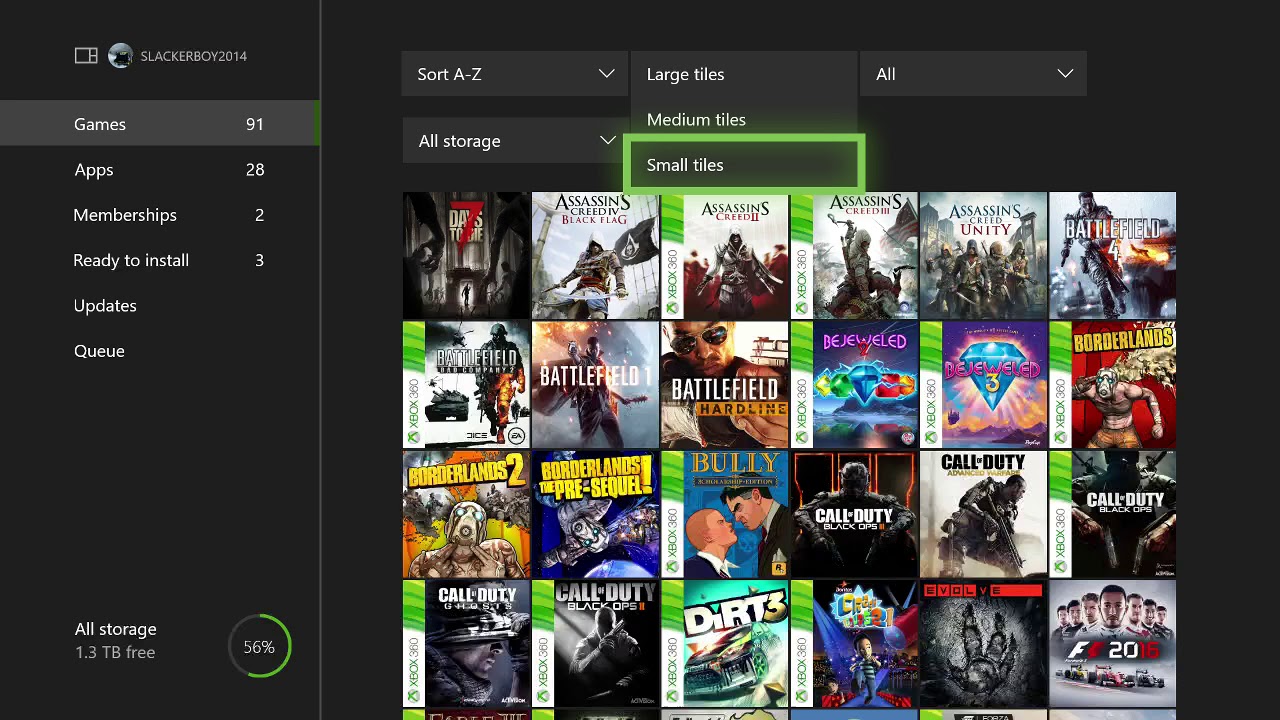This is a detailed screenshot of Slackerboy2014's game collection on their gaming console interface. The background features a gradient of gray and dark gray, divided into two distinct sections. On the right side, there is a narrow column displaying the username "Slackerboy2014" alongside an avatar icon. Below this, six interactive menu options are listed: Games, Apps, Memberships, Ready-to-Install, Updates, and Queue. The Games option is currently highlighted, revealing that Slackerboy2014 has 91 installed games.

Further down this right section, there is additional information indicating the storage status. It is reported that out of the total available storage, 1.3 terabytes are free. Adjacent to this information, a percentage dial is visible, featuring a green bar that is slightly over halfway filled, showing 56% of the storage is utilized.

Dominating the left and center of the screen, an array of game tiles showcases the variety of installed games. Slackerboy2014 has selected the 'Small Tiles' viewing option, which enables the display of 24 colorful game icons at once, providing a comprehensive snapshot of their game library.